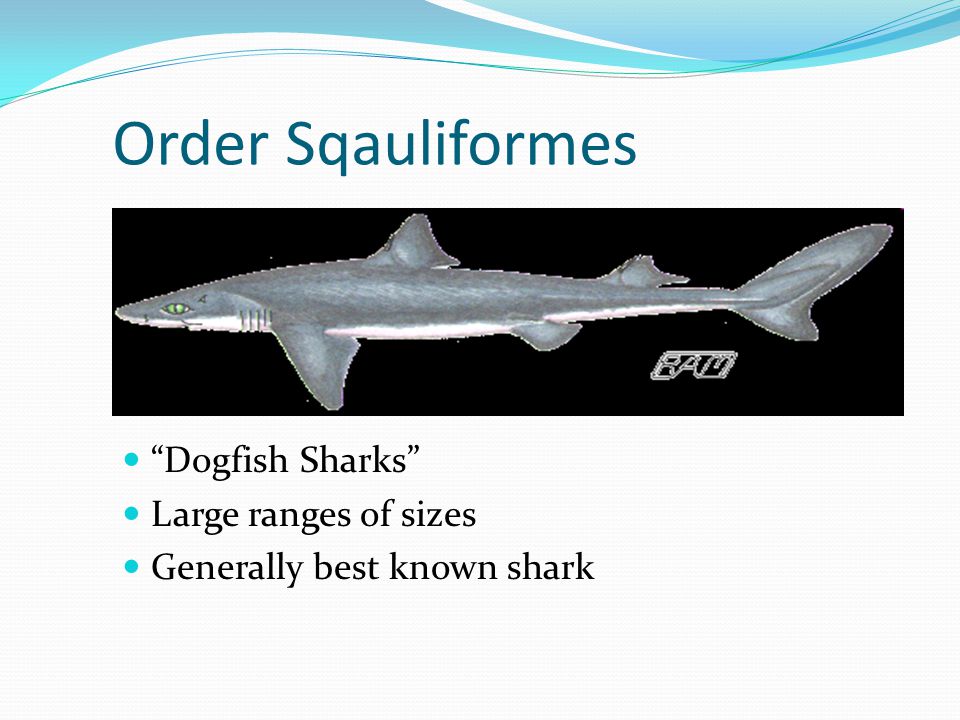This image, resembling a PowerPoint slide utilized for educational purposes, illustrates a sleek, gray shark with green eyes and a white underbelly, swimming towards the left within a dark black rectangle. Titled in large teal letters at the top, "Order Squaliformis," it provides a scientific context for the shark. Above the title, a wavy blue design evokes the ocean, enhancing the aquatic theme. Below the image, three turquoise bullet points succinctly inform viewers: "dogfish sharks," "large range of sizes," and "generally best known shark." The overall slide features an off-white background with subtle vertical and horizontal lines, suggesting a professional presentation format. Small, likely creator initials are faintly visible, adding a personalized touch.